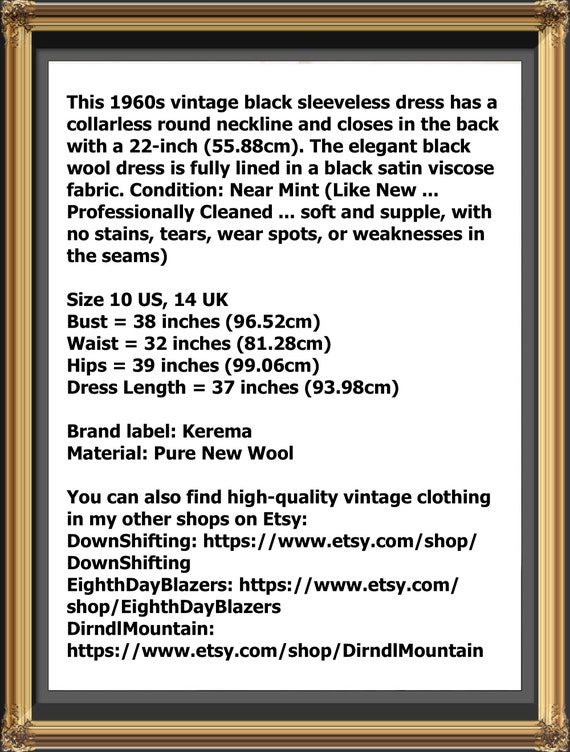This photograph showcases a rectangular, gold-framed informational plaque set against an off-white background. The plaque features black text detailing a vintage black sleeveless dress from the 1960s. The dress boasts a collarless round neckline and is designed to close at the back with a 22-inch (55.88 centimeters) zipper. Made from elegant black wool, the dress is fully lined with black satin viscose fabric. The condition of the dress is near-mint and presents as virtually like new, having been professionally cleaned. The material remains soft and supple, free from any stains, tears, wear spots, or weaknesses in the seams. This dress is a size 10 U.S. (14 U.K.), with a bust measurement of 38 inches (96.52 centimeters), a waist of 32 inches (81.28 centimeters), hips measuring 39 inches (99.06 centimeters), and a total dress length of 37 inches (93.98 centimeters). It features a brand label from "Karima," and the material is noted as pure new wool. The plaque also provides several web addresses where potential buyers can find more information online.